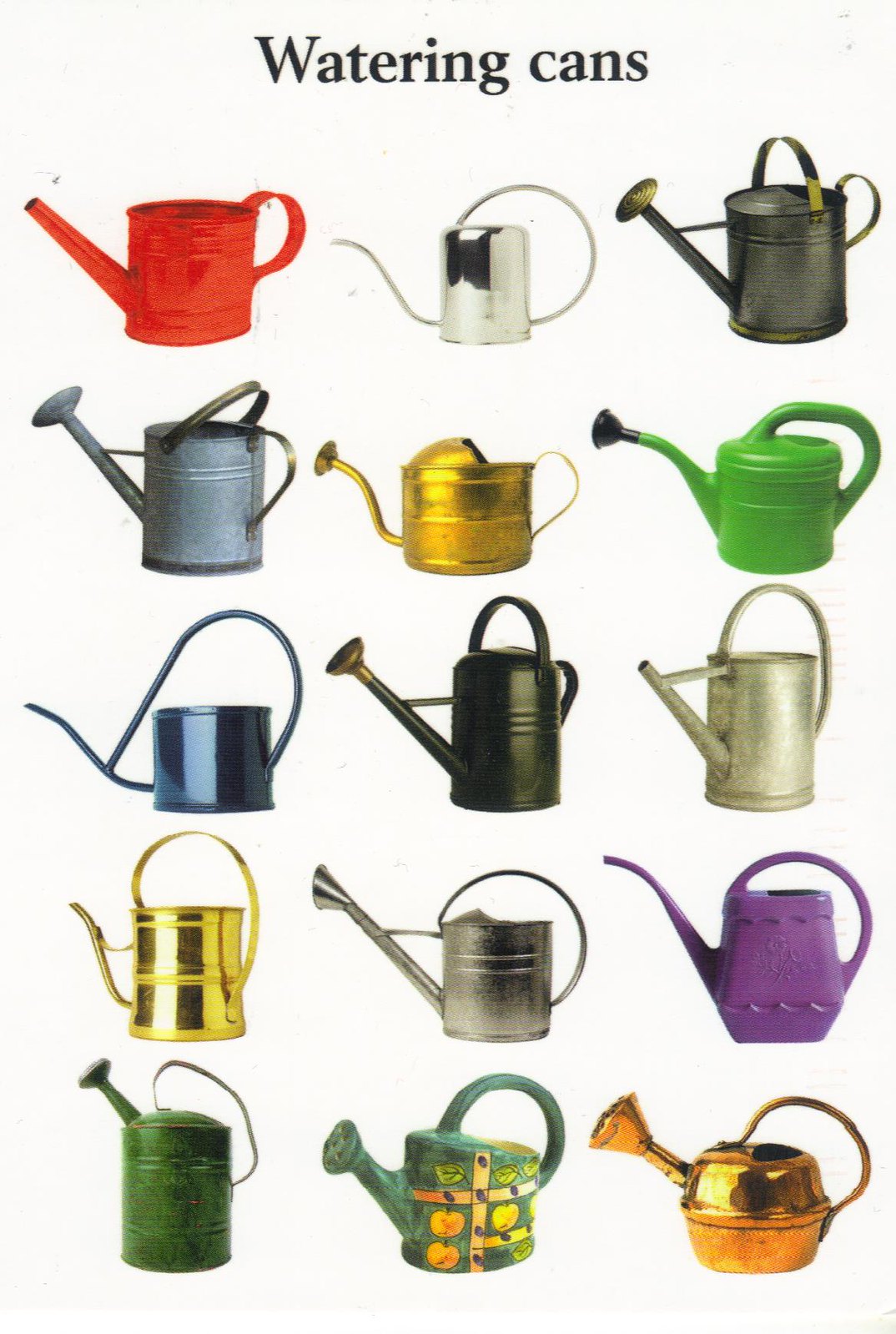The image displays a diverse collection of 15 watering cans arranged against a stark white background. At the top, in bold black letters, it reads "Watering Cans." These cans vary widely in design, color, and material. Some are made of plain, unadorned metal, while others are whimsically colored or have a rustic appearance. The arrangement is in a grid-like fashion, three cans across and five cans down.

Starting from the top left, the cans range from a red one with a matching handle to a silver one, followed by a black can with gold accents. Below them, a green can with a black tip is next to an entirely gold can. Further down, there is a light blue can with gold handles, situated near another light blue can. A black one with a gold tip is centrally positioned, with a silver one and a purple one flanking it on the right. In the bottom row, there is a green can with a design featuring oranges, apples, and green leaves, beside a plain green can and a golden one.

The collection includes cans made from stainless steel, aluminum, and various types of plastic. Some have strainers on their spouts, while others do not, indicating different functionalities. The overall presentation suggests a display possibly intended for a website or a commercial catalog.